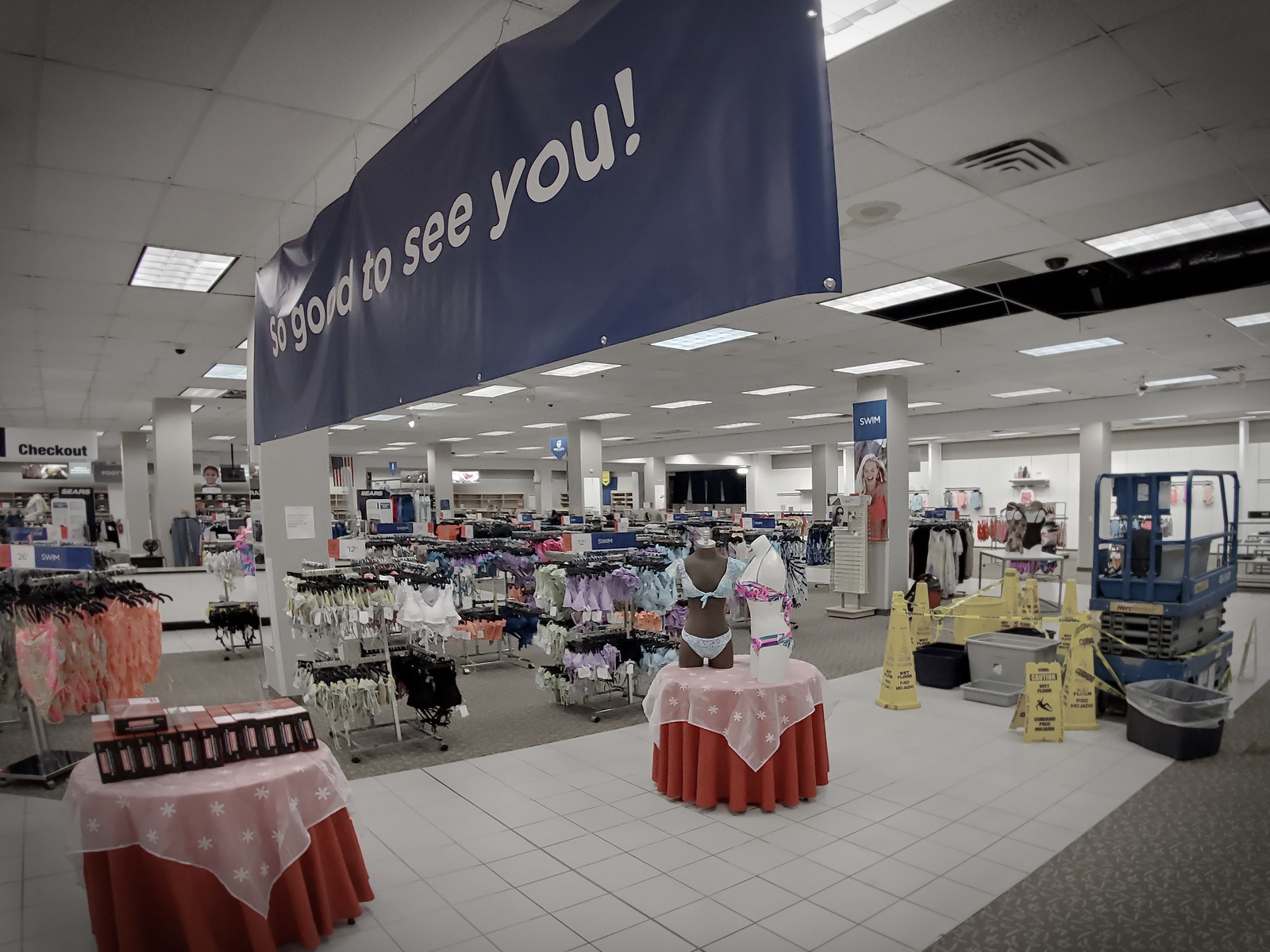The photograph captures a large, brightly lit department store, reminiscent of a Marshalls or TJ Maxx, specifically showcasing the women's lingerie and swimwear sections. Dominating the scene is a large, blue banner at the top with the white text, "So good to see you!" The ceiling features recessed fluorescent lights and fans. The store floor includes gray carpets and gray ceramic tiles, and various racks and display tables filled with colorful lingerie in shades of purple, red, white, blue, orange, and pink. 

In the top left corner, there is a "Checkout" sign, while a "Swim" sign is situated near the center top. The display tables in the walkway are draped with long, floor-length orange tablecloths overlaid with white lacy ones, and they hold mannequins without arms, legs, or heads, modeling baby blue and floral bikinis. Toward the right of the lingerie section, there are yellow caution signs, yellow tape, and a blue apparatus indicating maintenance work. The ceiling panels appear removed in some areas, possibly due to a water leak, with buckets placed on the floor to catch dripping water. The overall ambiance is stark due to the white-painted walls and the harsh, bright lighting.